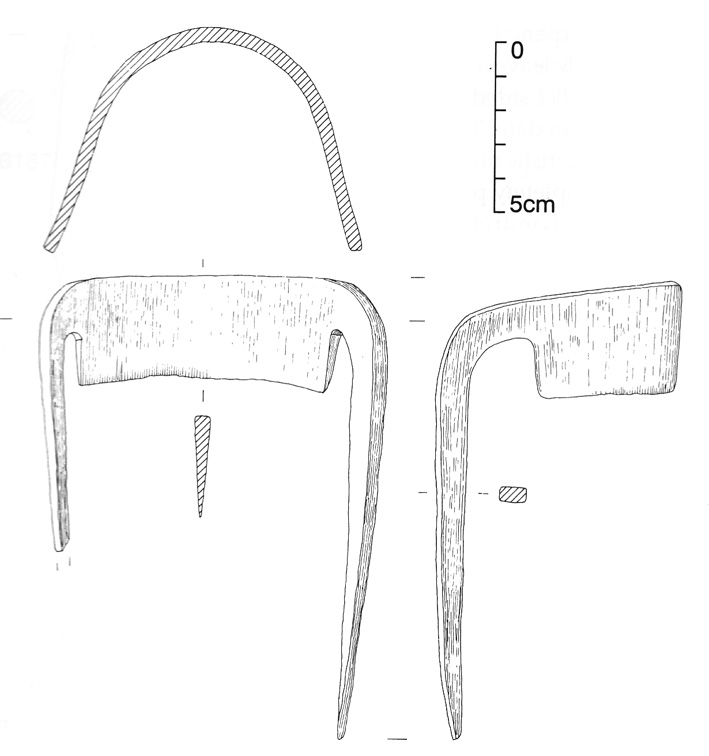This black and white diagram features a series of metal objects, each uniquely shaped and arranged for measurement purposes. Along the top right-hand side, there is a number scale ranging from 0 to 5 centimeters, indicating the dimensions of the objects. The first item at the top resembles a bent steel wire or rope, forming a half-oval shape above a larger object. Below this is a nearly square piece of metal with a spike protruding from its right side and a distinct, horn-like protrusion in the center. To the right of this, there is a smaller object that appears to be a partial mirror image of the larger square object with a curved design, forming its own unique structure. This detailed illustration provides multiple perspectives on various metal instruments, emphasizing their distinct geometries and possible functionalities.